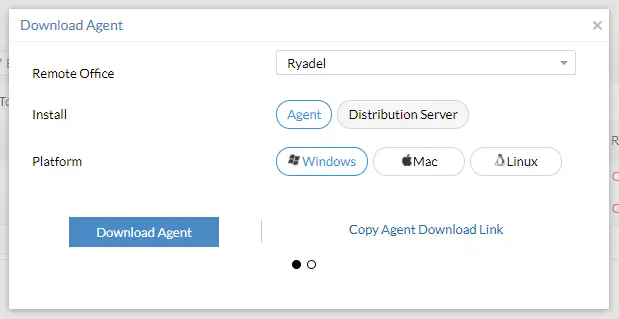The image depicts a white, horizontal rectangular pop-up box with a light gray border, set atop another section of a website. The box is translucent, allowing the underlying page to be partially visible. In the upper left-hand corner, the text "Download Agent" is displayed in blue font. Situated in the top right corner is an "X" for closing the pop-up.

The pop-up box is divided into various sections. Below "Download Agent," there are three subsections listed: Remote Office, Install, and Platform. Further down the pop-up, a prominent blue horizontal button labeled "Download Agent" is displayed.

On the right side of the box, a drop-down menu at the top reads "Riadel," with a downward arrow indicating additional options. Below this menu are five buttons labeled "Agent," "Distribution Server," "Windows," "Mac," and "Linux." Both the "Agent" and "Windows" buttons are highlighted with a blue circle and text, while the other buttons feature a white background with blue text.

Centered on the right-hand side, there is the blue link text "Copy Agent Download Link." At the bottom of the pop-up box, there are two circles: the left circle is filled in black, and the right circle has a black outline with a white center.